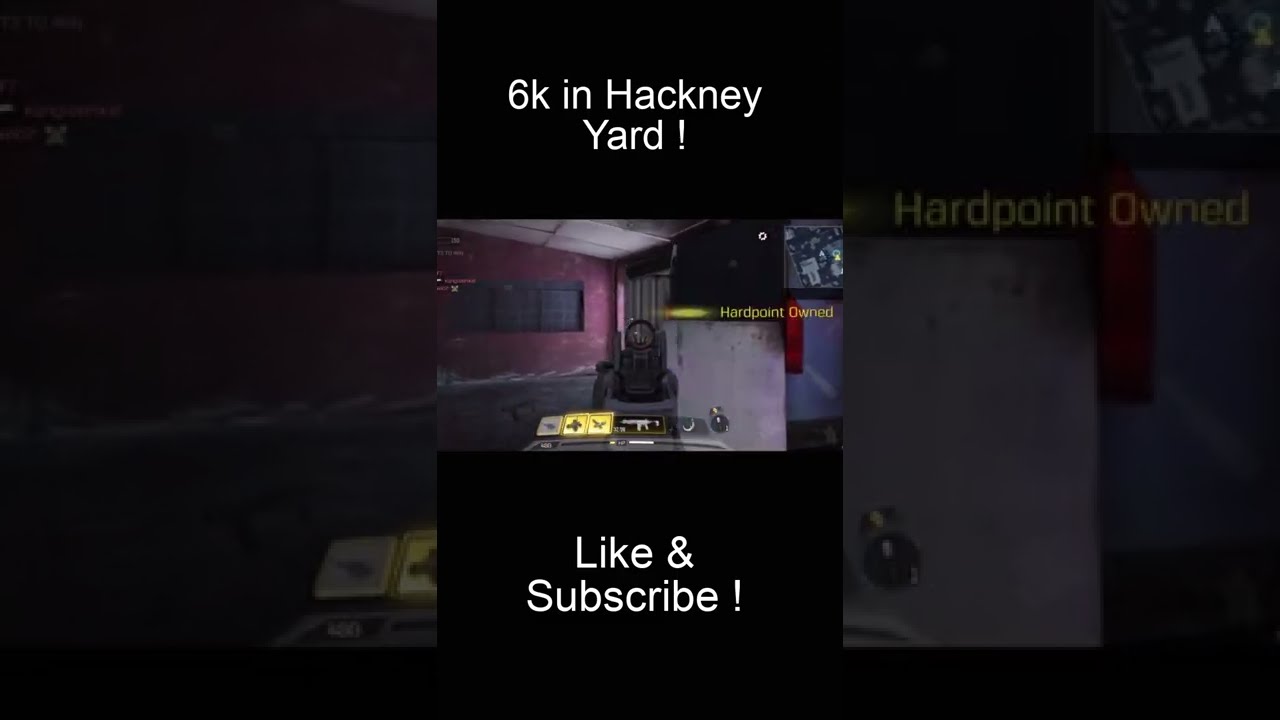This image appears to be a promotional screenshot from a first-person shooter video game, primarily set against a black background. At the top, white text reads "6K in Hackney Yard," and at the bottom, it prompts viewers to "Like and Subscribe!" with an exclamation point. The primary focus of the image is a central screenshot depicting a dimly lit in-game scene featuring a red wall with black windows and a dark floor. In the foreground, a black silhouette that resembles either a vehicle or robot is noticeable. Superimposed text within this central image indicates "Hardpoint Owned" in yellow font, accompanied by a yellow flash toward the left. Below the game scene, an icon with yellow squares and what appears to be a gun is visible. Additionally, the left and right sides of the main image display zoomed-in portions of the game scene, with the left side highlighting the in-game icons and the right side focusing on the "Hardpoint Owned" text. The entire visual is complex, featuring various colors such as yellow, burgundy, white, black, gray, and a hint of blue, all contributing to its intricate and immersive presentation.